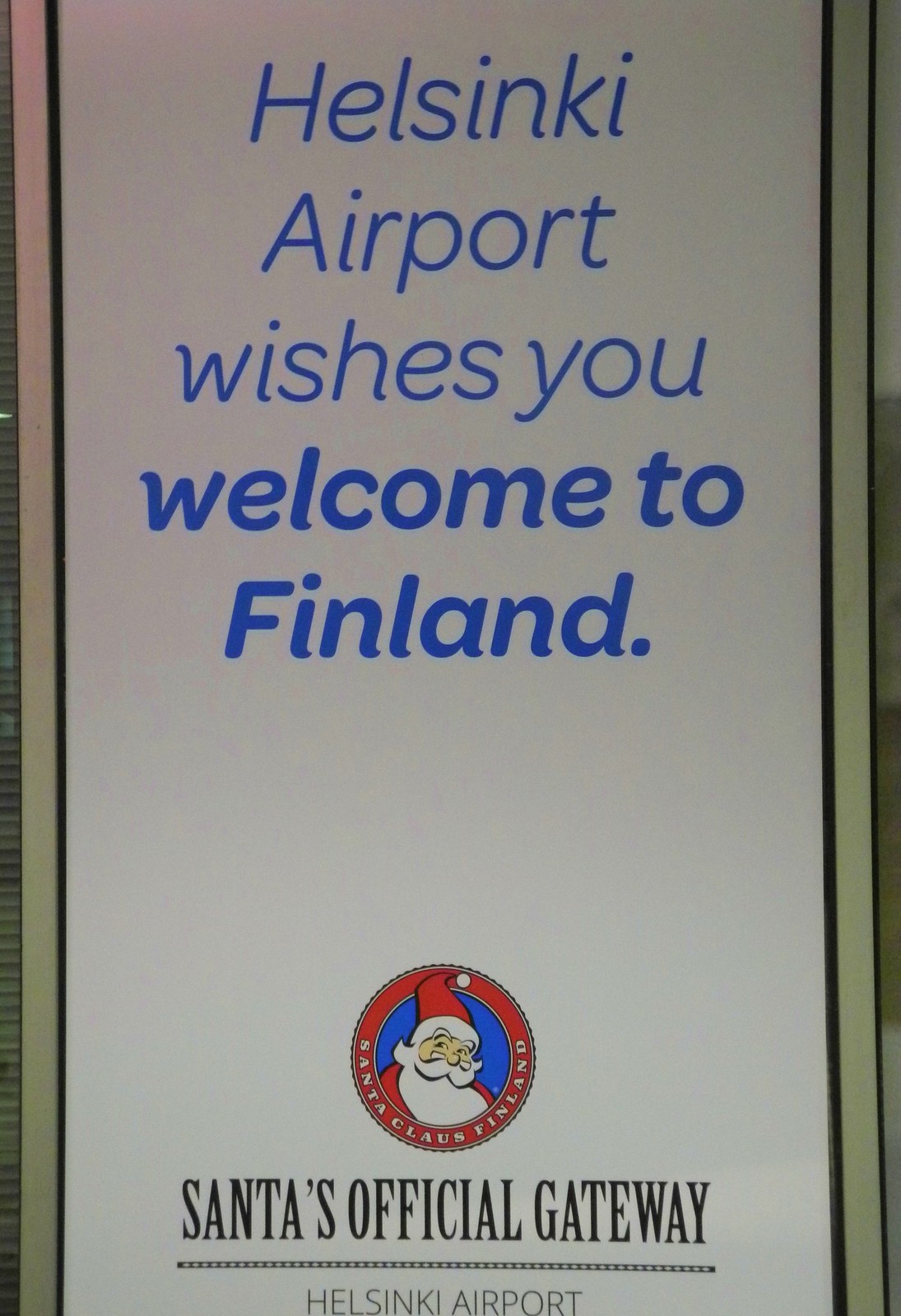The image depicts a festive poster or banner against a white background, likely taken indoors near a window with a drawn shade visible to the left. The main text in blue font reads, "Helsinki Airport wishes you welcome to Finland," with "welcome to Finland" emphasized in a bolder style. Below this, in black letters, it states, "Santa's official gateway Helsinki Airport." This is accompanied by a circular logo featuring a cartoon image of Santa Claus: he wears a red coat, red hat with a white cuff and ball, white beard, mustache, glasses on the bridge of his nose, and is set against a blue background. The logo is bordered by a cutout red circle with the text "Santa Claus Finland" around the edge. The poster is enclosed within a black border and appears to be a Christmas-themed decoration, aimed at bringing holiday cheer to travelers and visitors at Helsinki Airport.